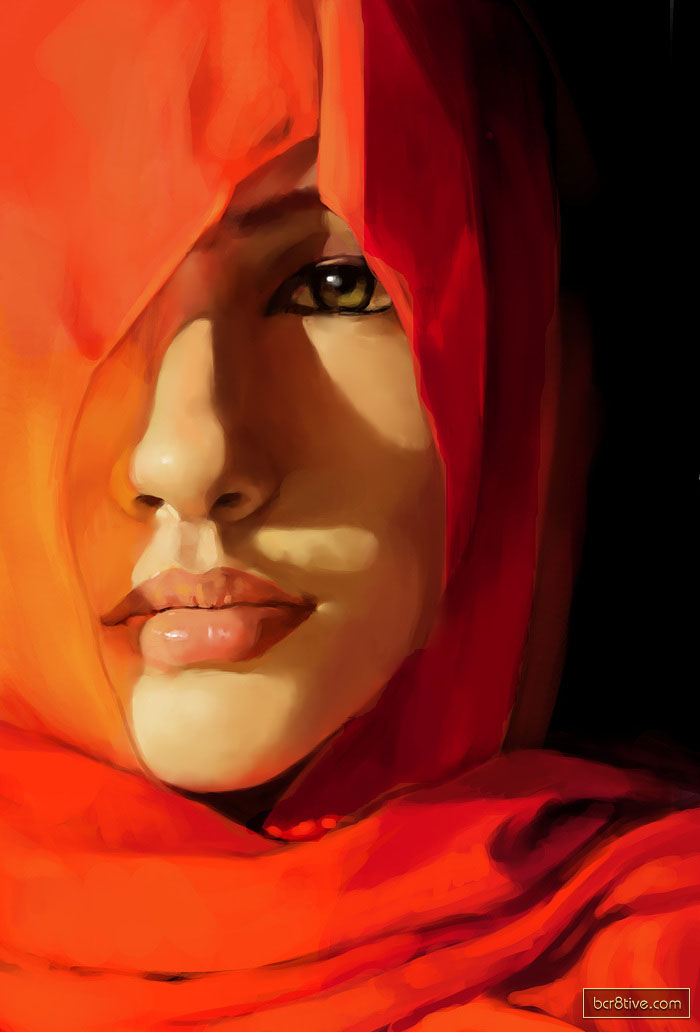The image depicts a striking drawing of a woman from the shoulders up, adorned in a red outfit. The fabric, a rich reddish-orange, drapes elegantly around her, showcasing intricate folds highlighted with dark accents. The background transitions from a deep black on the right to a vibrant red and orange on the left, creating a dramatic contrast. This fabric covers her left eye entirely, leaving only her expressive right eye visible. Her right eye, accentuated with black eyeliner, gleams a vivid green. Her lips are painted a soft pink, and subtle shadows play across her face, adding depth to her delicate features.